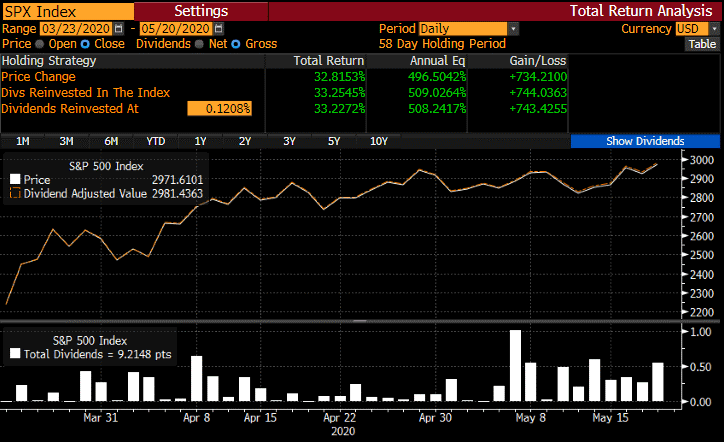This image is a detailed chart analysis of the S&P 500 index (SPX) displayed on a Bloomberg terminal, capturing data from March 23rd, 2020, to May 20th, 2020. The chart visually represents the price movement of the S&P 500 index along with the dividend-adjusted value during this period. Key metrics highlighted include a price change of 32.8153%, a reinvested dividend value of 33.2545%, and total dividends amounting to 9.2148 points.

At the top of the chart, there are sections dedicated to settings and analysis that outline annual equity returns and losses in USD. Below the chart, bars indicate volume data over time. The main graphical representation features a black background with an orange line that maps the index's performance. The chart shows a notable increase from a low of 2,200 points to about 3,000 points within the specified timeframe. This detailed visualization provides an insightful look into the market's recovery and performance during this pivotal two-month period.